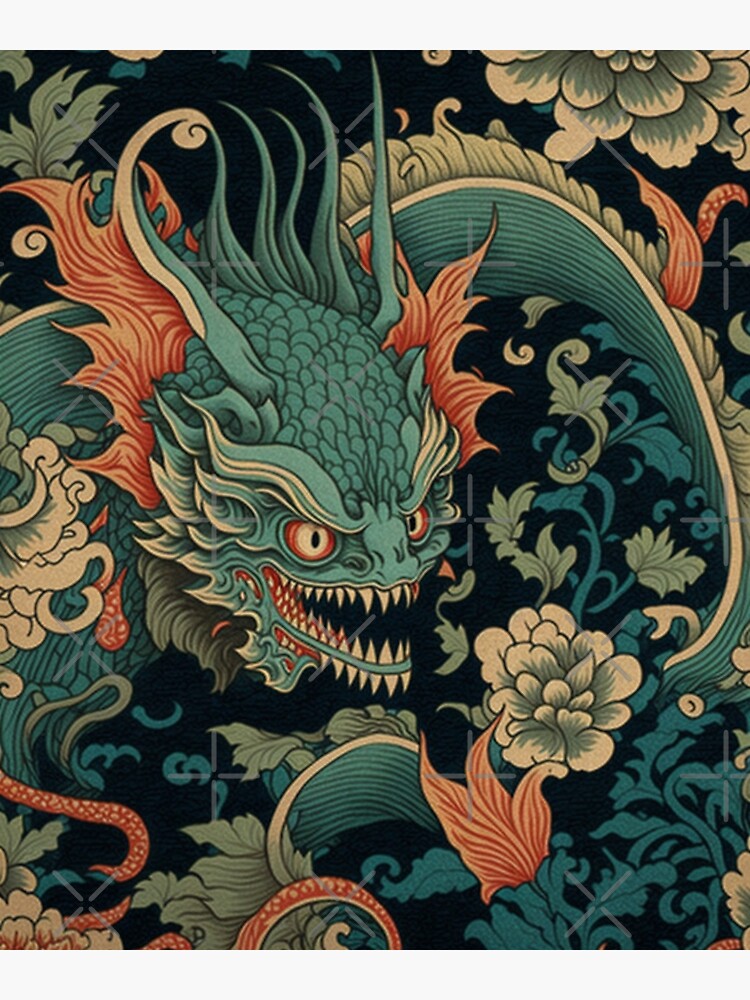The image is a contemporary, Japanese-style artwork depicting a very ornate and fiercely expressive anthropomorphic dragon. The dragon, primarily in shades of green and blue with red and tan accents, has a face filled with sharp teeth, including teeth under its mouth, and angry, wide-open red eyes that are directed towards the bottom right corner. Its open mouth and exposed teeth contribute to its menacing expression. The dragon's long body and tail flow abstractly through the piece, intertwining with an array of decorative plants, flowers, and vines that share its colors, creating a very busy and vivid scene against a black background. The flowers, in hues of light greens, blues, and whites, blend seamlessly with the dragon, making the boundaries of its form difficult to discern. The overall atmosphere of the artwork is a fierce portrayal of anger and mischief, with the dragon's presence dominating the intricate, colorful background.